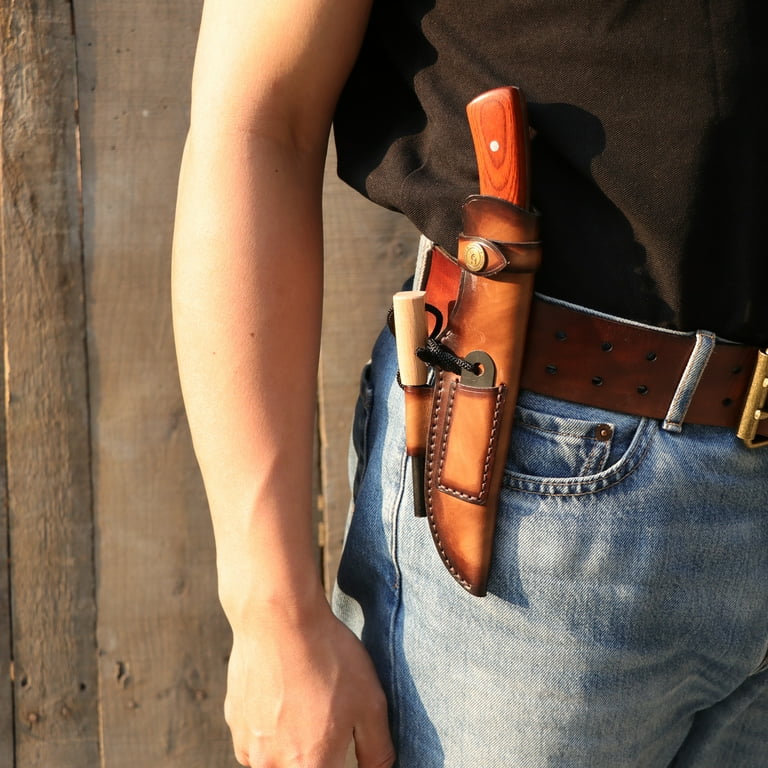The image features a side profile of a man modeling a bowie knife holster product for potential buyers. He is dressed in a black t-shirt and blue jeans, standing with his right arm resting naturally by his side. Affixed securely to his brown leather belt, which is adorned with a gold buckle, is a caramel-colored holster with darker edges designed to hold the bowie knife. The holster also includes a specialized attachment for a sharpening tool, which is predominantly wooden with a black blade and a convenient keyring. The bowie knife itself boasts a robust wooden handle, demonstrating its craftsmanship. The overall setup is intended to showcase the practicality and aesthetic appeal of the holster and its accompanying accessories.